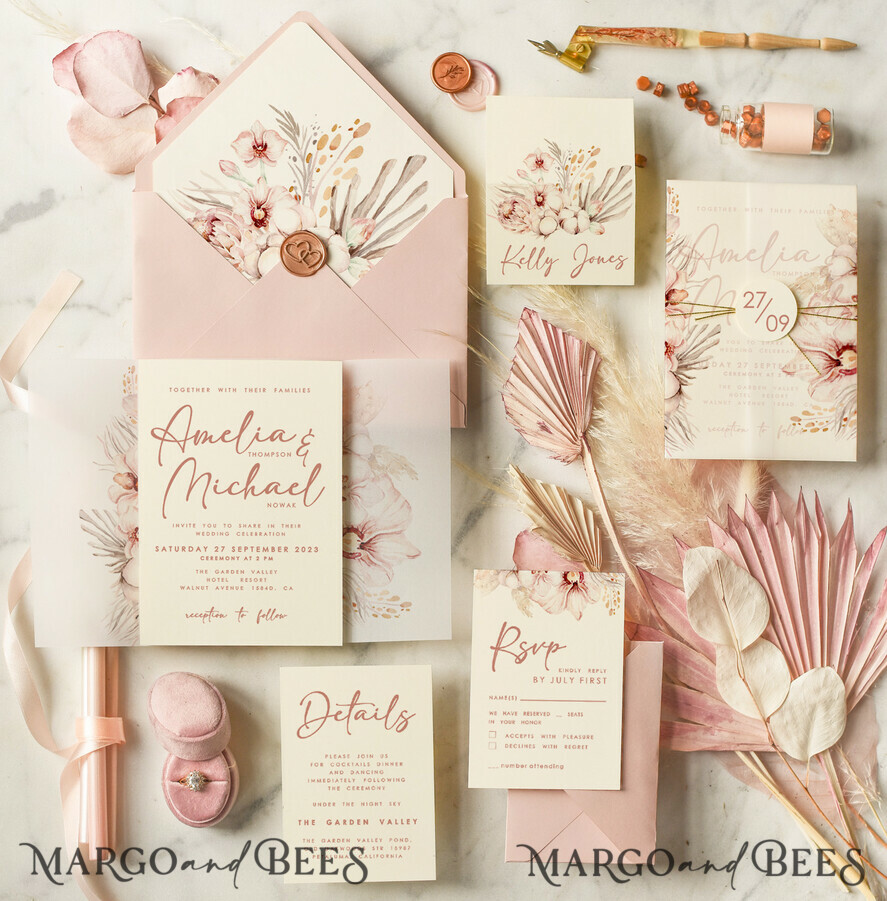This top-down photograph showcases an elegant array of wedding stationery set against a white marbled background. The color palette is predominantly soft pinks, whites, creams, and beiges, creating a feminine and delicate vibe. A variety of wedding invitations for Amelia and Michael are prominently featured, each adorned with intricate floral patterns, including light pink roses and wispy baby’s breath. The invitations are complemented by matching light pink envelopes. Detailed text includes the names Kelly Jones, Amelia, and Michael, and specifics such as the ceremony date—Saturday, September 27th, 2023, at 2 p.m.—and an RSVP deadline of July 1st. Floral watercolor designs with light green leaves enhance the overall aesthetic. At the bottom of the image, the text "Margot and Bees" appears twice, once on the left and once on the right, adding a branded touch to the ensemble.